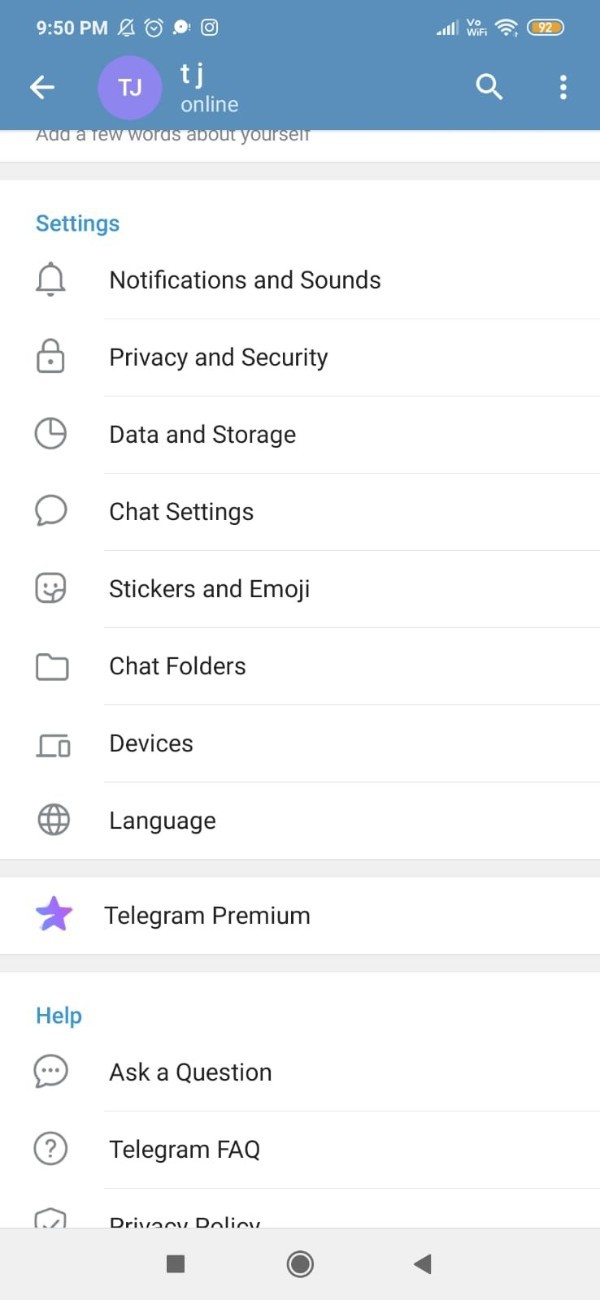This image is a cell phone screenshot of the Telegram app's settings panel. The screenshot is rectangular, being taller than it is wide, and seamlessly blends into the white background of the screen. 

At the top, a light blue horizontal rectangle serves as a header, displaying the time "9:50 p.m." on the left along with typical cell phone status icons on the right, including signal strength and a battery icon indicating a 92% charge. 

Within the main content of the screenshot, we see a user who is currently logged into Telegram, identified by a purple circle with the white initials "TJ," suggesting that TJ is online.

The settings tab is open, presenting various adjustable options listed in succession. These options include:
- Notifications and Sounds
- Privacy and Security
- Data and Storage
- Chat Settings
- Stickers and Emoji
- Chat Folders
- Devices
- Language

A thicker horizontal divider separates these from additional sections below.

Following this divider, further options are displayed:
- Telegram Premium
- Another horizontal divider
- Ask a Question
- Telegram FAQ
- Privacy Policy

At the bottom of the screenshot, there is a light-colored rectangle containing record, stop, and play buttons, likely related to the voice command or screen recording functionality.

Overall, this detailed screenshot showcases the settings interface of the Telegram app as accessed on a mobile device, providing a comprehensive view of the various configurable options available to the user.